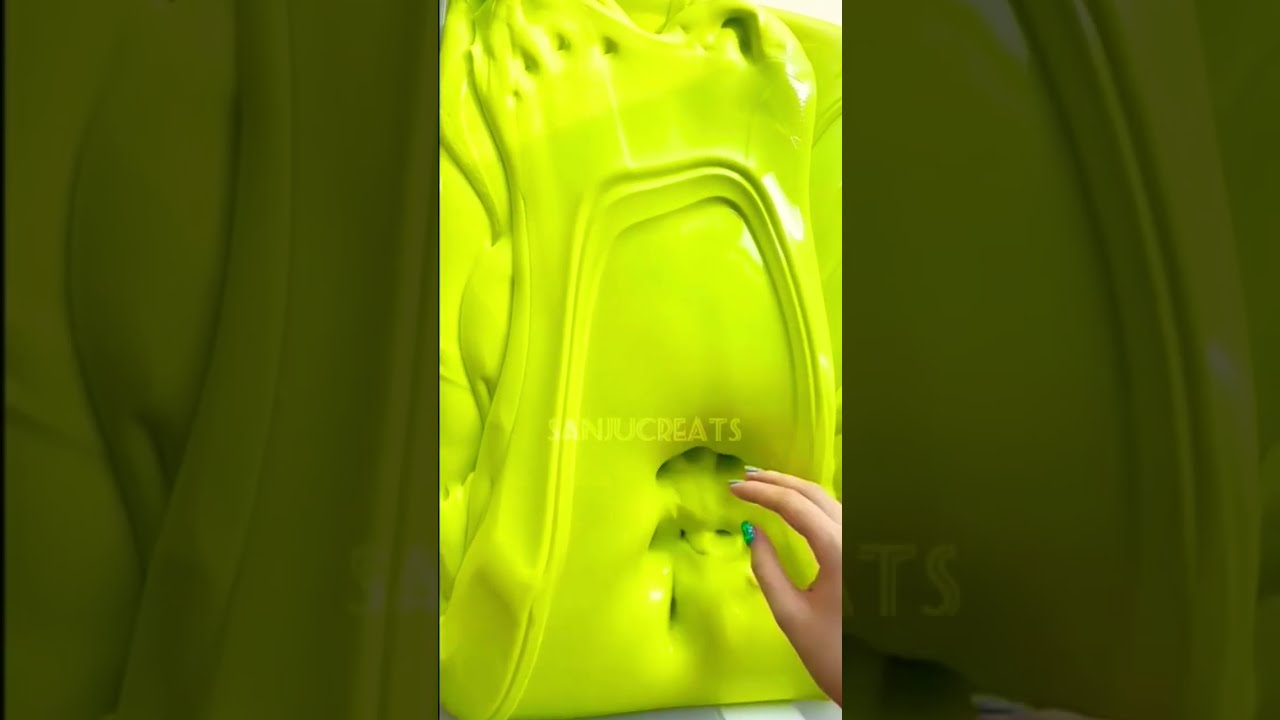The image is a horizontally-oriented rectangular picture divided into three vertical panels. The outer two panels are a dark olive green with vertical, wave-like striations, resembling a draped curtain extending from top to bottom. The middle panel is a stark contrast, featuring a lime green surface that resembles shiny Play-Doh, molded without a specific form but with a somewhat vertical design that arches from left to right and back down. You can see the indentations made by a hand, with fingerprints embedded into the lime green surface. A right hand, appearing from the bottom right corner of the middle panel, shows a white-skinned thumb bent slightly and the forefinger and middle finger curved, almost touching the thumb. The thumb is painted with bright green nail polish, while the other two fingernails have a paler color. Across the lime green surface in the middle panel, there is white capital lettering spelling "S-A-N-J-U-C-R-E-A-T-S." The left and right panels show the letters "T" and "S" near the bottom left side.